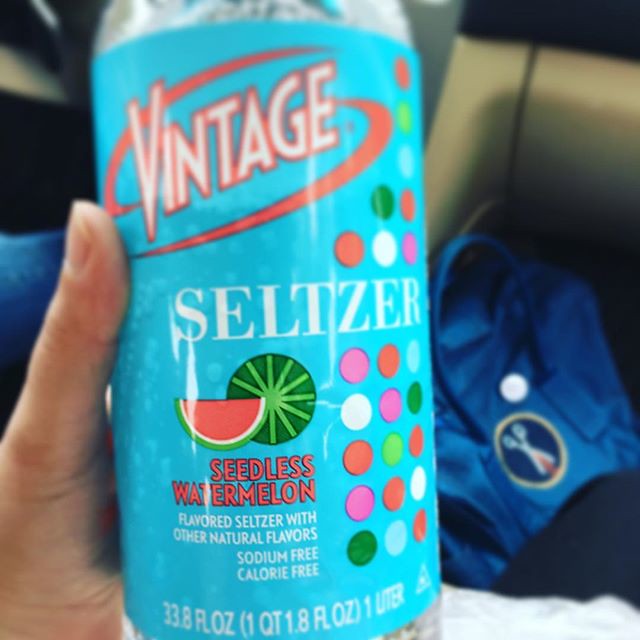A close-up image captures a person holding a blue aluminum can in their left hand, with the thumb partially visible on the left side of the frame. The can features intricate designs at the top and bottom, although these are partially cropped out of the image. The word "Vintage" is prominently displayed at an angle near the top of the can. Below it, assorted colorful dots—green, white, orange, and pink—decorate the left side, adding a vibrant touch. The word "Seltzer" is centrally located, partially overlapping the dotted pattern. Beneath this, the can displays images of watermelon slices, including both an end piece and a cut piece, with the label "Seedless Watermelon" written clearly underneath.